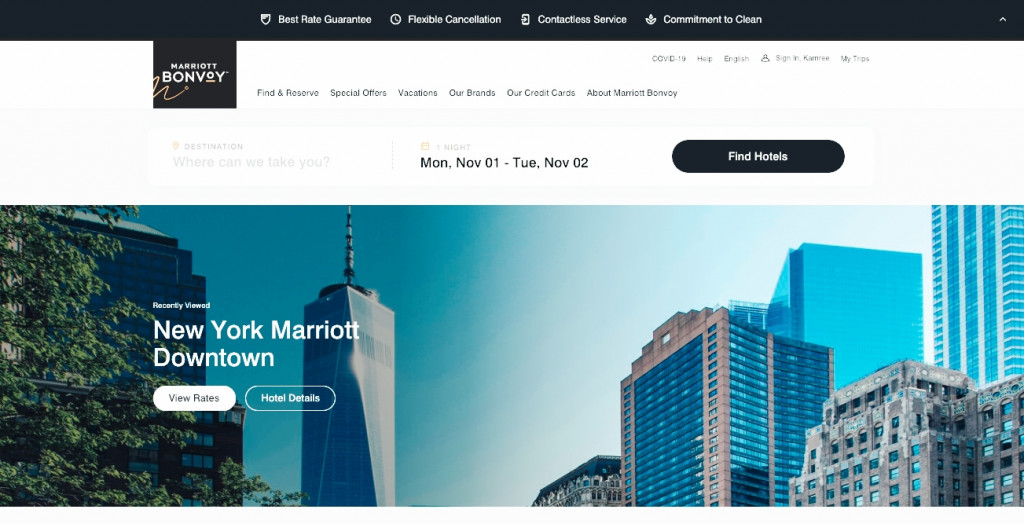This image is a screenshot of a hotel booking webpage, specifically for Marriott Bonvoy. In the top left corner, the Marriott Bonvoy logo is prominently displayed. The top part of the page features a thin black header bar with white text, offering service guarantees such as "Best Rate Guarantee" and "Flexible Cancellation." Below this header, a white section occupies approximately one third of the page, containing interactive boxes for selecting the location, dates, and the "Find Hotels" button.

The main content area showcases a large photograph of the New York Marriott Downtown, which fills a little more than half of the screen. Overlaying the photograph is a button labeled "View Rates" as well as a link to hotel deals. The webpage presents a structured layout designed to facilitate hotel booking, prominently featuring the brand and key functionalities.